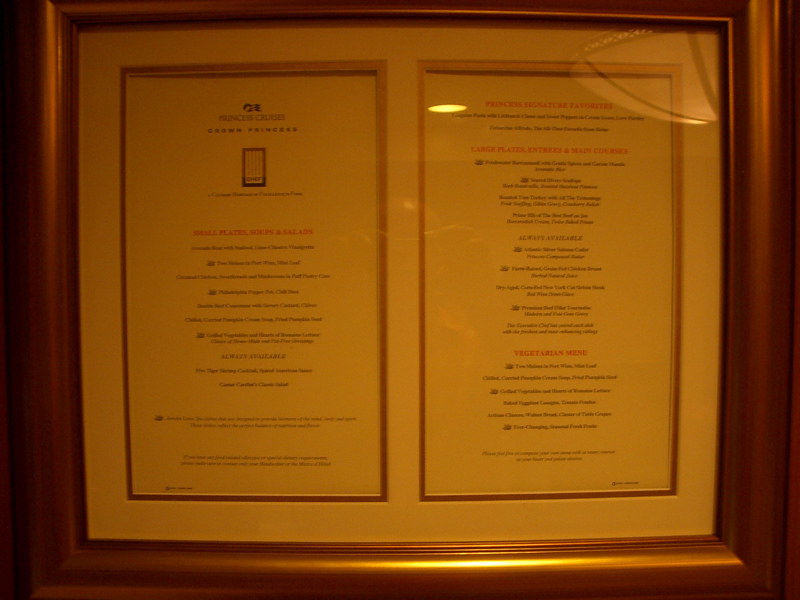The photograph captures a large, almost rectangular frame with a copper-like finish. Inside the frame, a white background is visible, which is further divided into two equal rectangular sections, positioned side by side with a gold-copperish border around each section. These sections appear to be some form of an announcement or a menu.

The section on the left-hand side features a small rectangular image at the top, followed by red lettering that seems to serve as a section title. Below the title, a list of items, possibly entrees or small plates, can be found, though the text is difficult to discern due to the darkness.

The right-hand section is divided into three parts, each listing different objects. However, the font is exceptionally small, making it nearly illegible in the photograph.